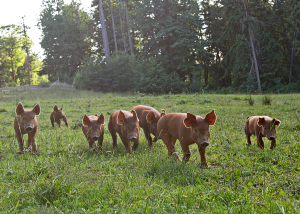This is a small, horizontal, rectangular image capturing a group of seven brown pigs in a grassy field. The green grass extends from the bottom to the middle of the image, with the pigs dispersed throughout this area. In the foreground, a large pig leads the way, followed by a line of five pigs—three clustered in the center, one on the left, and one on the right. A seventh pig trails behind, appearing smaller due to its distance from the camera. The pigs, with their big ears standing up straight and round bodies, are walking towards the camera, looking well-fed and at ease, possibly searching for food or heading home. The background features a variety of trees, including some lighter-colored deciduous ones on the left and taller, possibly evergreen trees filling the rest of the skyline. The upper left corner shows a patch of gray sky, adding a touch of brightness to the otherwise overcast scene. The serene setting suggests a peaceful midday moment in nature, devoid of any human presence.